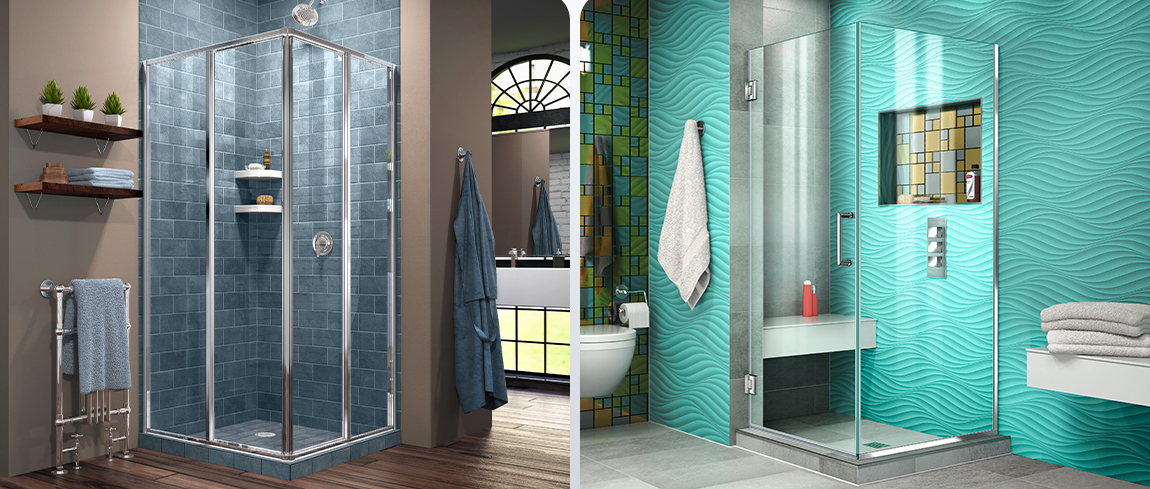The image presents a side-by-side comparison of two distinct bathroom styles. On the left, a sleek, sophisticated bathroom features a shower stall with gleaming blue subway tiles, enclosed by glass doors with stainless steel fixtures. The light brown painted walls provide a warm contrast. Adjacent to the shower, two wooden shelves are mounted: the top one adorned with small plants, and the bottom one holding neatly stacked towels. A silver towel rack is positioned to the left of the shower, and a bathrobe hangs on a hook to the right, completing the elegant setup.

The bathroom on the right exudes a more vibrant and bright ambiance with its textured bright blue wallpaper. The glass shower cubicle houses a white bench and showcases an eye-catching tile inlay composed of gray and light green tiles. This same tile motif is repeated near the toilet area, where part of the toilet bowl and the toilet paper holder are visible. A white bench with four white towels rests on the right side of the image, and a towel hangs from a hook beside the shower, adding to the clean and refreshing look of the space.